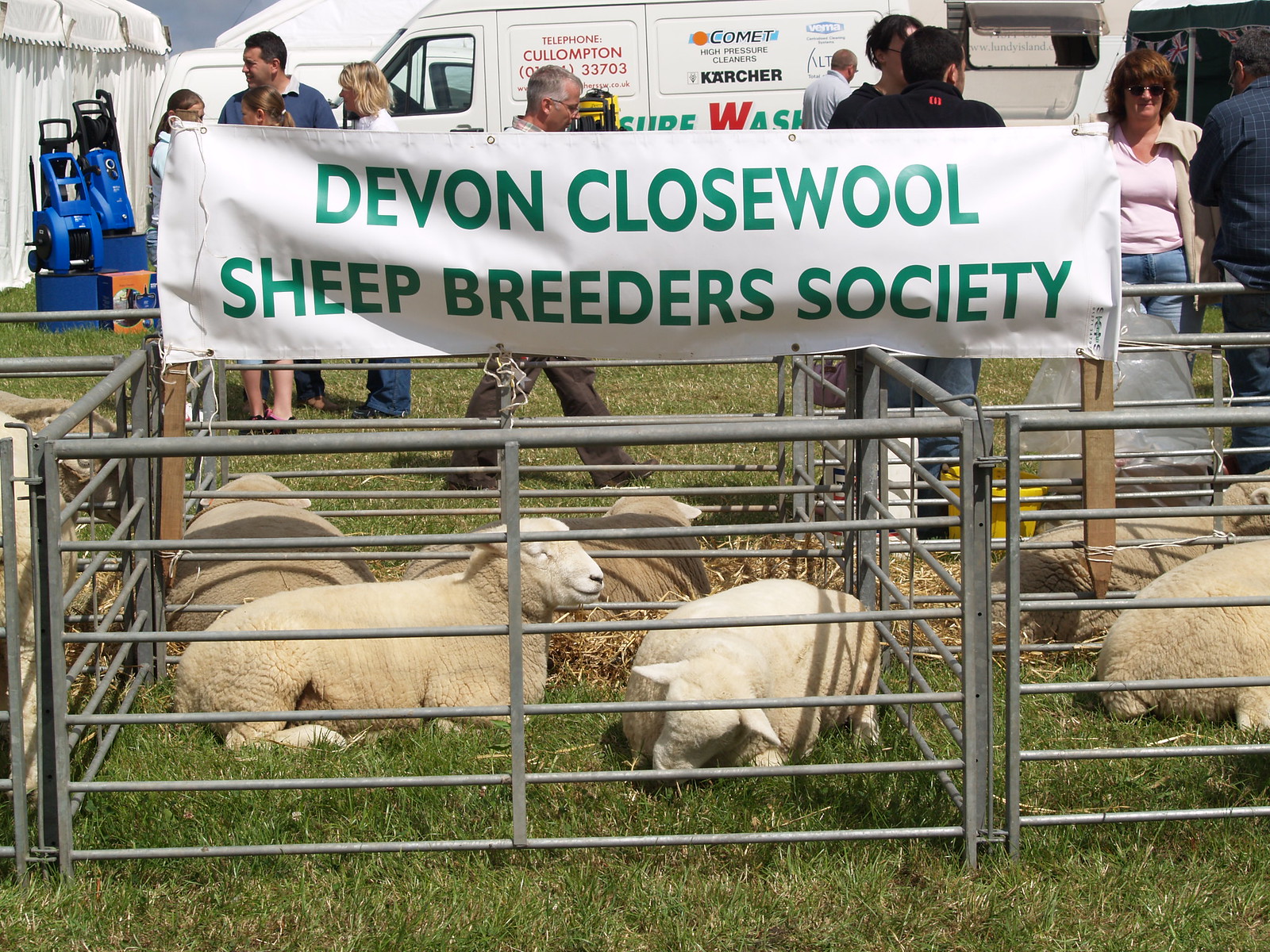This is a detailed color photograph capturing an outdoor festival or agricultural exhibition focused on sheep breeding. At the center of the photo, several metal pens contain various groups of sheep. The sheep in the forefront are white and appear to be resting or sleeping on the ground. Behind them, in a separate pen, are two brown sheep with their backs to the camera. In total, four or five steel pens are visible, each containing sheep. A prominent white banner with green text reading "Devon Close Wool Sheep Breeders Society" is attached to the pens with sticks. The background features white tents and a white panel van decked with promotional text advertising a Pressure Wash business in green, white, and red. Blue pressure washers are displayed on stands nearby. Various patrons—both men and women—are strolling about, including a woman in a pink shirt, jeans, and a cream-colored jacket with brown hair and sunglasses, conversing with a man in a dark blue shirt. They are surrounded by more people who appear to be evaluating or purchasing sheep and farming products.